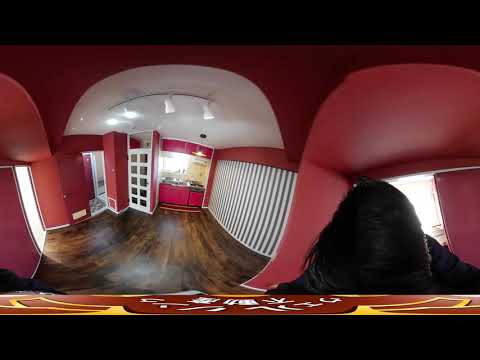A photograph captures a highly distorted image of a red room, likely taken with a wide-angle lens, contributing to the unusual perspective. The red walls dominate the space, punctuated by a striking painting and various white accents. At the top part of the ceiling on the left, a cluster of three tracking lights is partially illuminated—only two of the left lights are turned on, while the two right lights remain off. One wall on the right features vertical white stripes extending down to the dark hardwood floor, described as a mocha color. A curious red bar runs along the bottom of the image, adorned with white Chinese characters. The foreground includes the back of a person's head with dark brown or black hair, partially obscuring the view. Amid the room's red expanse, there are white elements such as a door and part of the ceiling. Although the exact layout is unclear due to the image's distortion, hints of a kitchen-like area with a stove and sink near a doorway can be discerned.